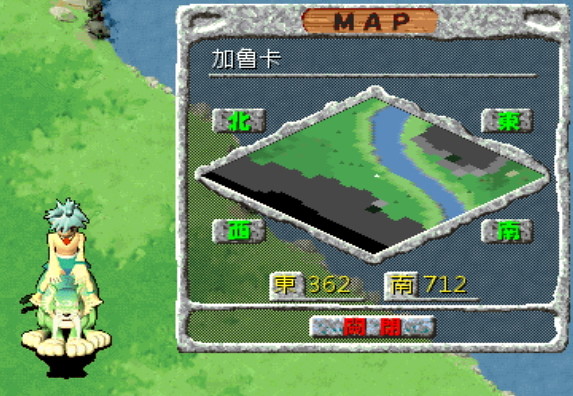This detailed image from a video game screen features a focused square on the right-hand side, outlined in gray with a wooden area at the top. The word "MAP" is clearly displayed in black letters on the wooden strip. Beneath the label "MAP," Asian characters appear in gray against a cornflower blue-gray background. The central diagonal image within the square is the map itself, showing various stone-like squares around its perimeter, each marked with Asian characters and numerical values, 362 on the left and 712 on the right, in yellow.

The background of the map includes partially visible water in the upper right corner and a green shoreline on the left. Positioned at the bottom left of the image is an anime-style character resembling a figure from Dragon Ball Z. This character stands on a dark pedestal, accompanied by a small dog. Another visible figure is straddling a large green wolf with white feet. This second character is dressed in yellow, has brown skin, green hair, a red mask over his nose and mouth, and appears to have his head bowed. The entire scene combines detailed gaming elements with lush greenery and vivid water imagery.